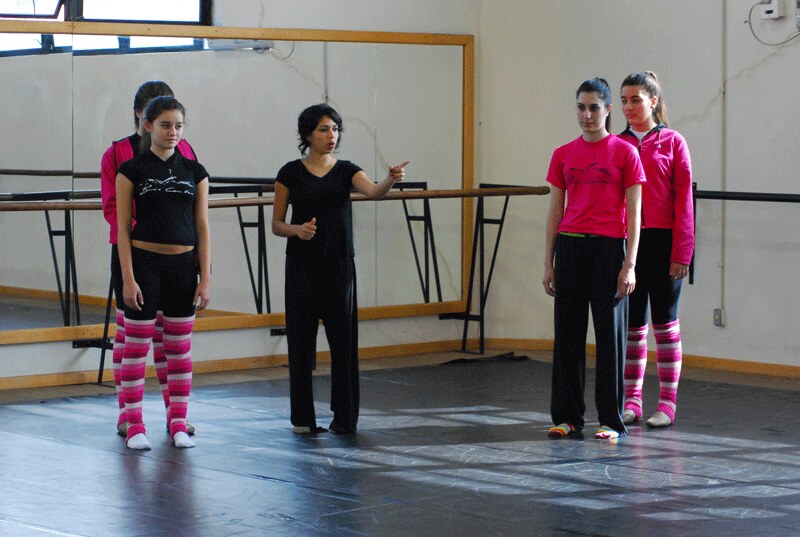The image depicts five women standing in what appears to be a gymnastics area or a dance studio with matted flooring that seems to be either dark green, dark blue, or black. The central figure, presumably the instructor, is clad in a black shirt and black workout pants. 

Flanked to her left, from the observer's perspective, are two women dressed in white and pink leggings; one of them, positioned in front, is further identifiable by her black shirt and shorts. The woman behind her is mostly obscured. On the right side of the instructor, from the observer's viewpoint, are two more women dressed in pink tops—one in a t-shirt and the other in a long-sleeve shirt. 

The room features white walls and is adorned with mirrors and a ballet barre along the back wall. Reflective surfaces capture windows toward the top left corner of the image. The majority of the women are wearing black bottoms, and some have distinctive socks: three with high pink striped socks and another with rainbow socks. All appear to be focusing on the instructor, who is gesturing off into the distance.